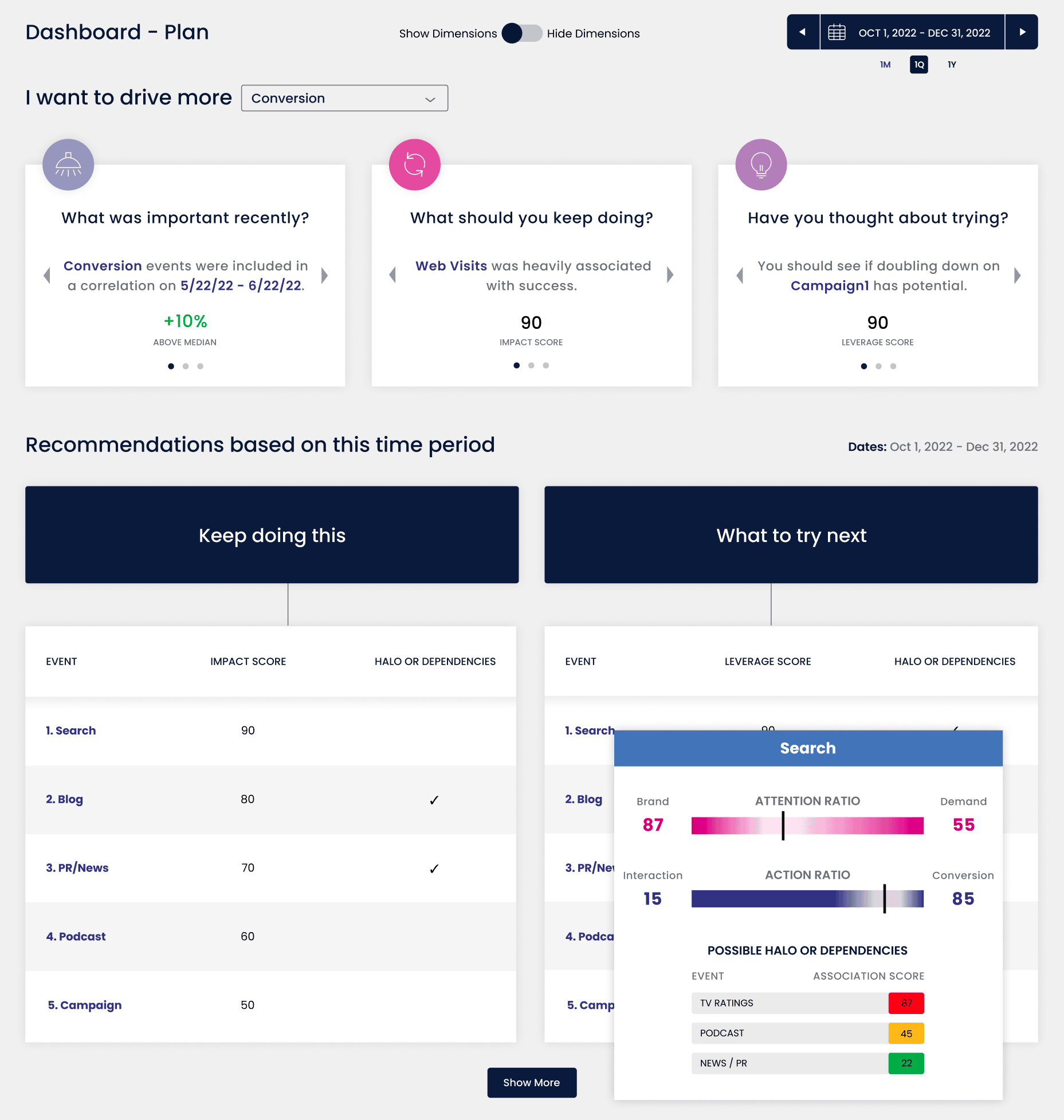This image is a screenshot displayed on a light gray background. At the top of the screenshot, there is a header in either black or navy blue text that reads "Dashboard - Plan," with both the 'D' and 'P' capitalized. Below the header, there are options to "Show Dimensions" and "Hide Dimensions," with "Show Dimensions" currently selected.

Underneath these options, there is a drop-down menu labeled "I want to drive more," with "Conversion" selected from the menu. On the right side of the screenshot, there is a calendar displaying the date range from October 1st, 2022 to December 31st, 2022. The calendar also indicates options labeled "1M," "1Q," and "1Y," with "1Q" (one quarter) being selected.

To the left, there are three distinct white sections containing information:
1. "What was important recently" – This section mentions that conversion events were included in a correction from May 22, 2022, to June 22, 2022, resulting in a +10% increase above the median.
2. "What should you keep doing" – This section highlights that visits were heavily associated with success, achieving a 90 impact score.
3. "Have you thought about trying" – This section suggests using the data to determine if doubling down on Campaign One has potential, with an average score of 90.

Further down, there are recommendations based on the time period specified (October 1st, 2022 to December 31st, 2022). Accompanying these recommendations are two banners:
1. "Keep Doing This" – This section includes the event impact score and mentions any halo effects or dependencies.
2. "What to Try Next" – This section outlines events and their respective scores, along with any halo effects or dependencies.